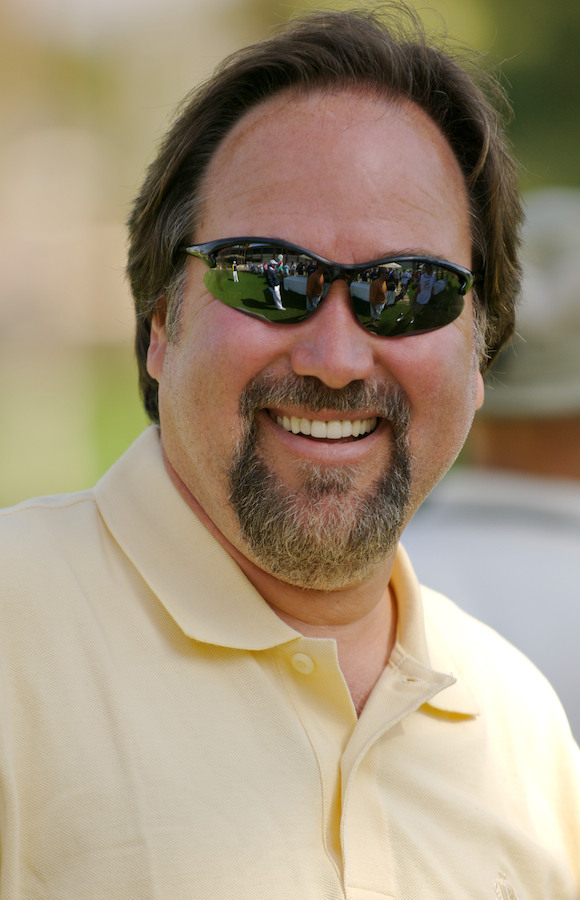This vertical, rectangular photograph captures a white man who appears to be in his late 40s to early 50s, wearing a light yellow collared button-down shirt. He has brown hair with a receding hairline, a mustache, and a close-shaven beard. His eyes are concealed by black sunglasses, which are reflecting a scene that suggests he might be at a golf game. The man is smiling broadly, showing his teeth, and he looks directly at the camera. The background is a blurred mix of yellow, green, and a bit of white. The image evokes a sense of familiarity, with the man bearing a resemblance to the character Al Borland from the show Home Improvement. The photograph shows him from the chest up, without his arms or hands visible.